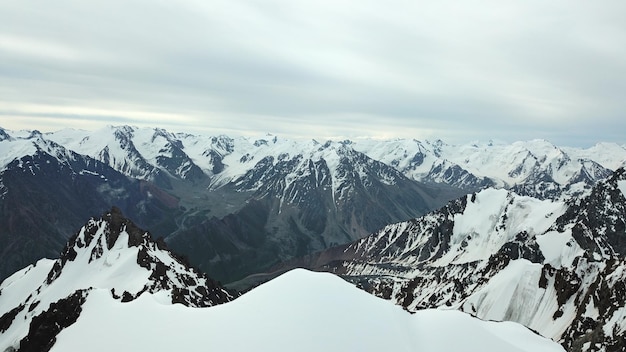This breathtaking photograph showcases a vast mountain range covered in pristine, white snow, juxtaposed with patches of exposed brown and black rock. The snow appears fresh, suggesting a recent snowfall. The image, taken in landscape orientation, captures multiple rows of snow-capped peaks and the deep valleys in between, which are dry and devoid of snow. The fore and mid-ground are dominated by these majestic mountains, extending into the background where the overcast sky appears heavy with clouds, casting a grayish-white hue over the scene. Some sunlight filters through but is largely obscured by the thick cloud cover, preventing the landscape from being fully illuminated. The overall tone of the photograph is a striking black and white with a subtle blue tint, and the image appears slightly overexposed. There are no signs of human presence or structures, emphasizing the untouched, raw beauty of this natural, panoramic scene.